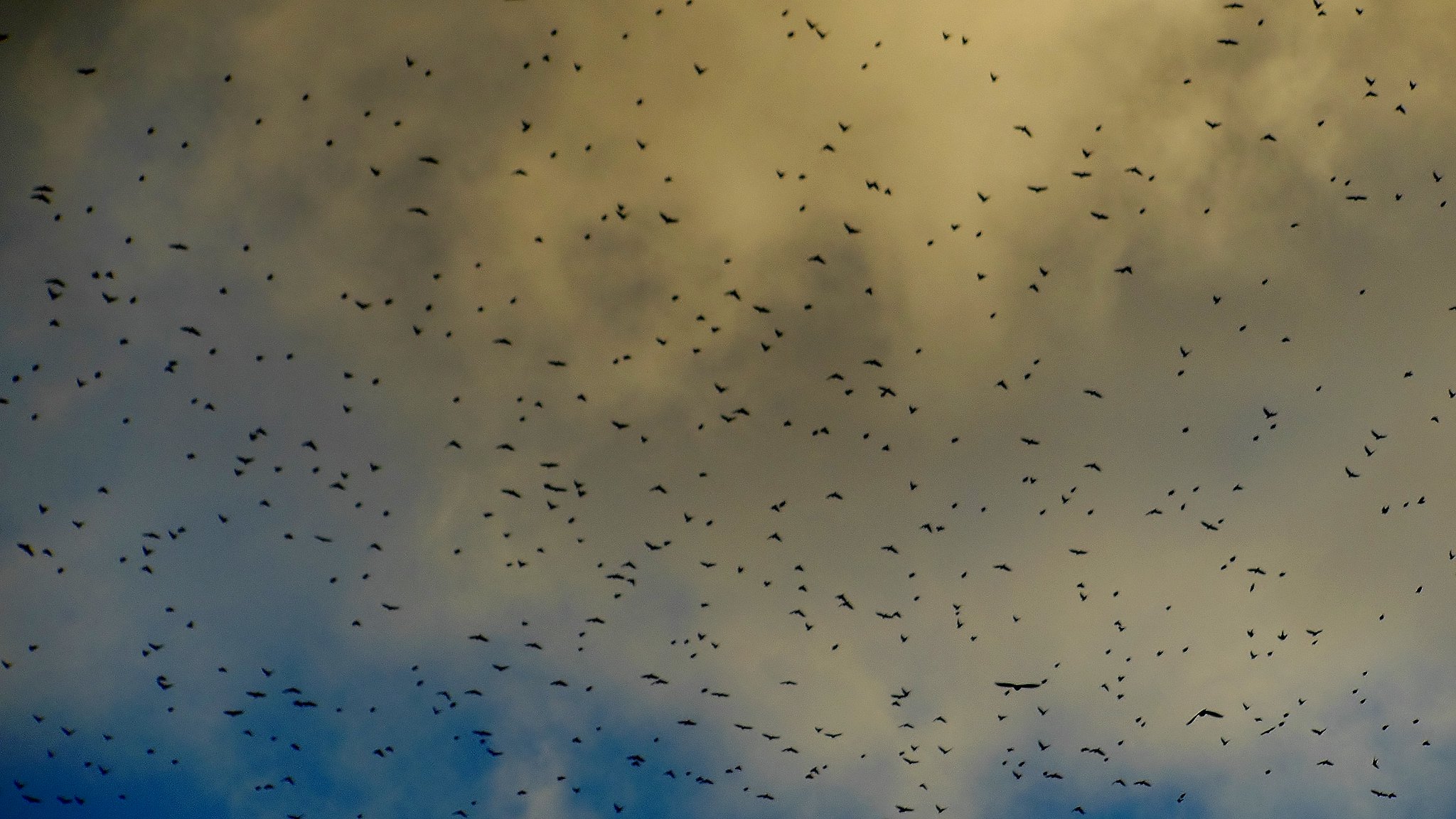This image captures an outdoor scene focused on a vast, cloudy sky featuring hundreds, if not thousands, of tiny black silhouettes scattered throughout. The sky is filled with different sized birds, possibly bats, their forms peppered across the expanse from the top to the very bottom of the photograph. The clouds range from white to light gray at the top right, gradually transitioning to darker shades, even bluish black, towards the bottom left. A small patch of dark blue sky peeks out from the bottom, adding depth to the scene. Despite the varying intensities of light and cloud cover, the tiny, winged creatures are a constant, moving aimlessly without any discernible pattern, creating an almost chaotic yet mesmerizing display.